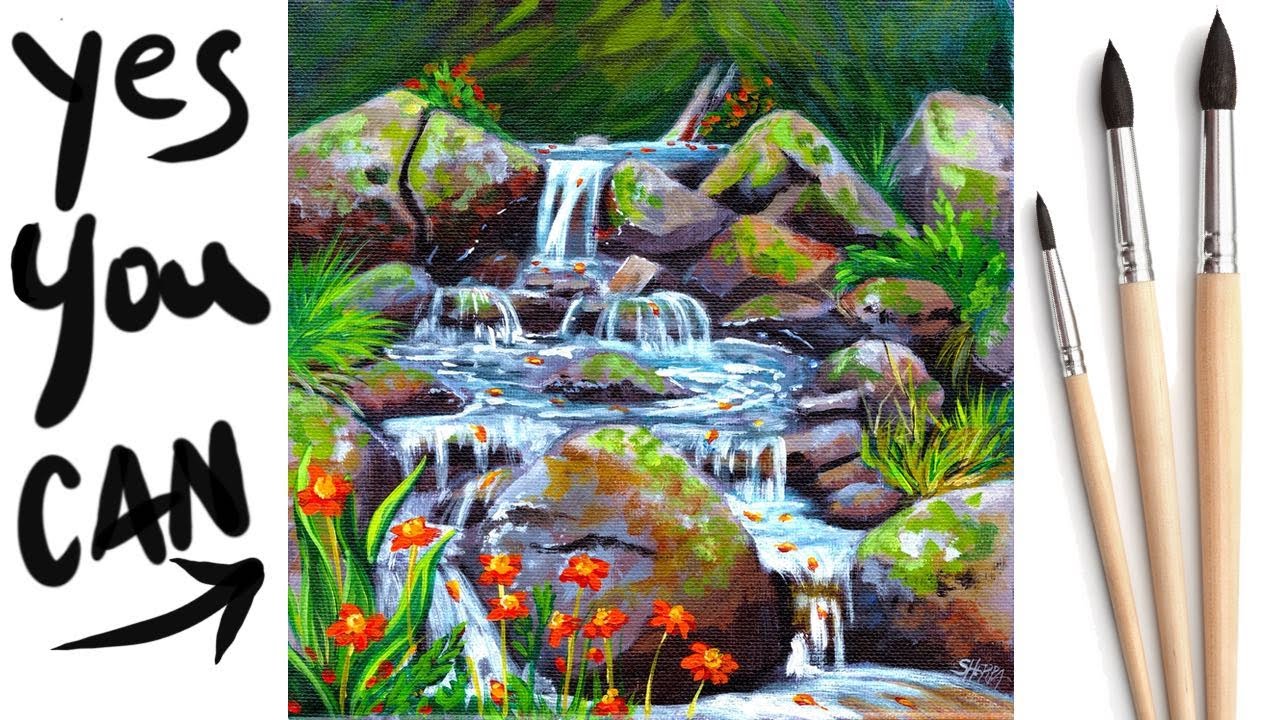The image features a detailed painting at its center, depicting a serene outdoor scene where a cascading waterfall flows down layered rocks into a creek surrounded by lush plants and vibrant flowers. The foreground of the painting showcases orange and yellow flowers, while the rocks are adorned with moss and little red flowers nestled at the bottom left corner. To the left of the painting, in bold black letters, the motivational text "yes you can" is displayed, complete with an arrow pointing towards the artwork. On the right side of the image are three paintbrushes of differing lengths, arranged from shortest to tallest from left to right. The brushes are clean, with black tips, and contribute to the overall artistic theme of the scene. The colors in the painting include a harmonious blend of orange, green, black, off-white, yellow, and blue, capturing the essence of a beautiful, tranquil, daytime garden setting.